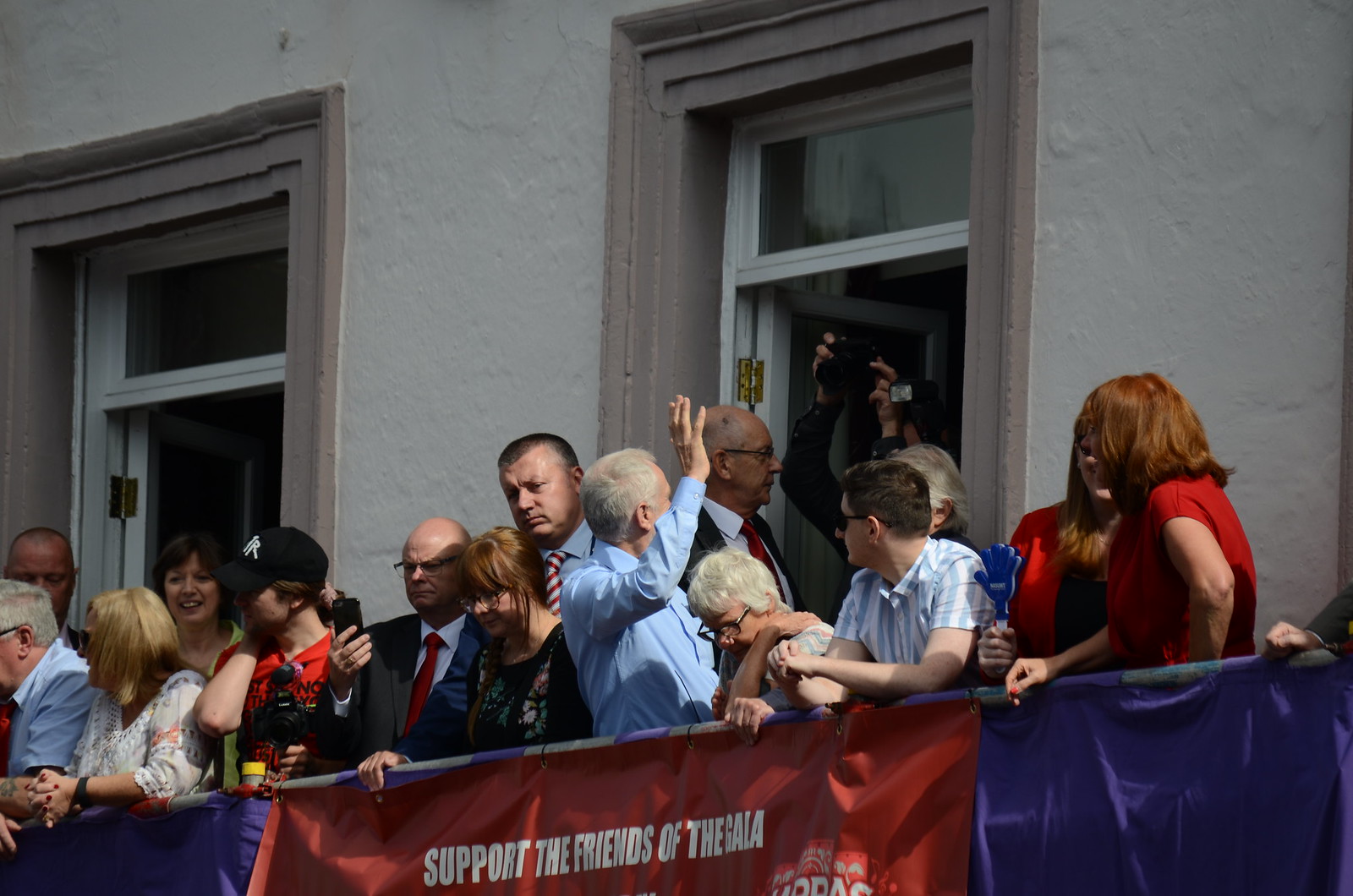The photograph captures a bustling scene on a balcony attached to the side of a white, textured building. Prominently, there are two purple banners and a central red banner reading, "Support the Friends of the Gala" in white text, draped over a guardrail. The balcony teems with approximately 15 to 20 people, including men and women dressed in varied attire—suits, ties, short-sleeved shirts, long-sleeved shirts, blouses, T-shirts, and even a baseball cap. A woman in a red dress stands out among the crowd, looking away from the camera. Another gentleman, sporting a short-sleeved shirt and sunglasses, casually leans on the railing. A man in a blue long-sleeved shirt is seen facing a central window, waving at a person inside who is holding a camera above their head. This central window, flanked by two openings that resemble doors, adds to the dynamic scene as it catches the focal activity of the gathering. The diverse group exhibits a mixture of poses—some are looking off the balcony, while others face different directions, contributing to the lively and somewhat celebratory atmosphere of the photograph.